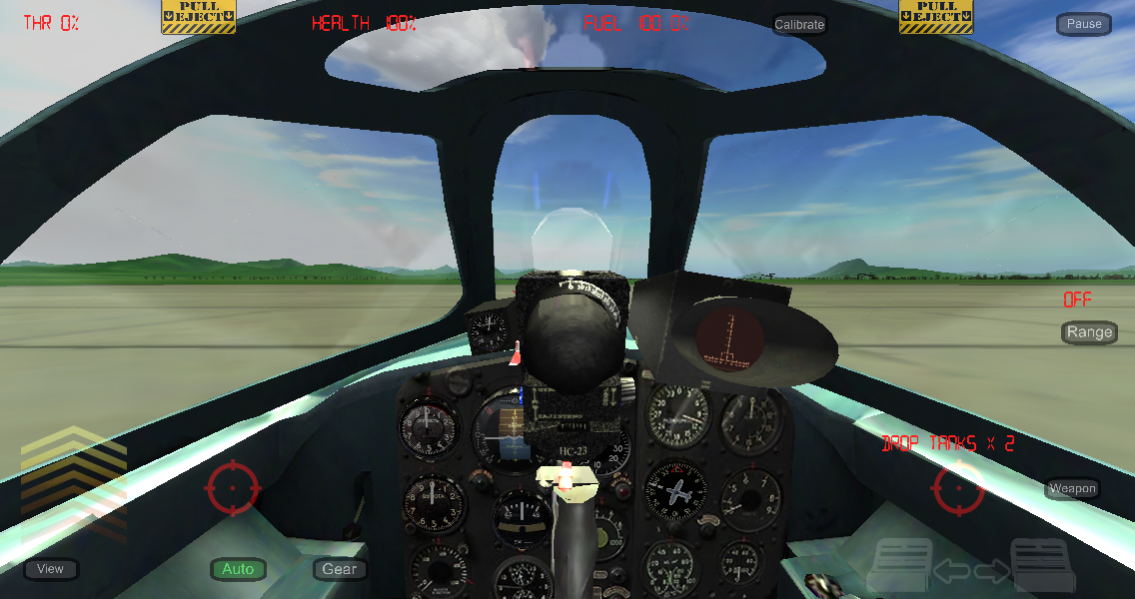This image depicts an incredibly detailed first-person perspective of a modern fighter jet cockpit, which appears almost like a high-fidelity video game simulator. The cockpit is equipped with an array of sophisticated controls, including numerous dials with white hands, a central joystick, and detailed instrumentation panels. The numerous dials—three on the left, six on the right, and five in the center—indicate various metrics such as compass readings, pressure, and speed.

The cockpit windows, encompassing a center window, side windows, and a top window, offer a panoramic view. Through these windows, a vivid horizon is visible, featuring low-riding green mountains and a blue sky dotted with clouds. The tarmac below the aircraft is tan-colored. Additional on-screen elements include text like "throw 0%," "eject," "health 100%," "fuel 100%," "calibrate," "off-range weapon," and "drop tanks," indicating various simulation or gaming features.

Noteworthy details such as the coordinates in the right corner and various pedal markers underscore the complex realism of the simulation. With the lush green mountains and clear skies ahead, the overall scene marries a technical cockpit environment with a picturesque, yet intense, landscape.